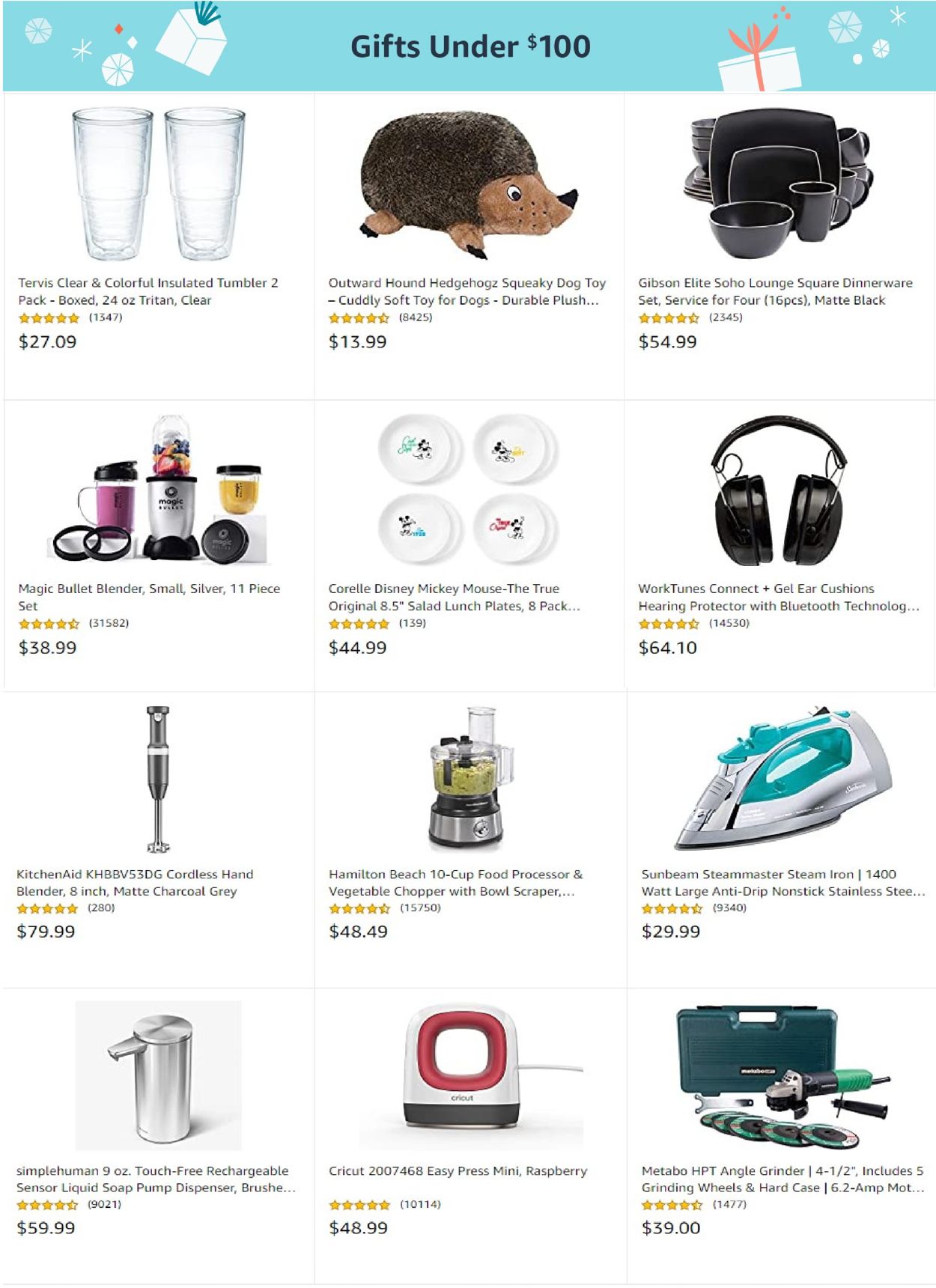The image depicts a vibrant shopping web page advertising "Gifts Under $100." The page features a prominent blue banner decorated with an envelope, snowflakes, and a white present adorned with a red bow, adding a festive touch. The web page showcases an assortment of items, starting with a set of clear glasses, specifically Tervis clear and colorful insulated tumblers, highlighted with a star rating and reviews tallying approximately 1,300, priced at $27.09. 

In the center, a hedgehog-shaped squeeze toy is available for $13.99. Nearby, a 16-piece kitchenware set is listed at $54.99. Further down, other items include a Magic Bullet blender, a set of dishes, and headphones. Additional products include a grinder, a cricket presser, an iron, rechargeable hand sanitizer, a food processor, a whisk, and more headphones. 

The layout organizes the products into four rows, with three items per row, totaling twelve diverse gift options. The webpage closely resembles an Amazon format, though its origin isn't explicitly stated. The array of items and potential lightning deals suggest a well-curated selection for budget-conscious shoppers.